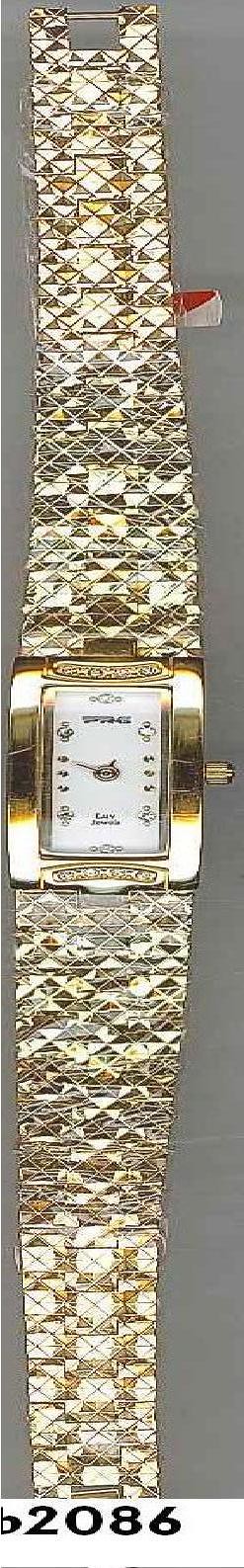The image features an elegant wristwatch set against a gray background with a white strip at the bottom labeled "B2086" in black writing. The timepiece is primarily gold, with a rectangular vertical watch face bordered by a smooth gold edge. The centerpiece of the watch has a white backdrop adorned with various logos and design elements, although the brand name remains illegible. The clock hands and the adjusting knob on the right side of the watch are both golden. The wristband is composed of a series of interlocking square and geometric shapes, adding an intricate and sophisticated element to the design.